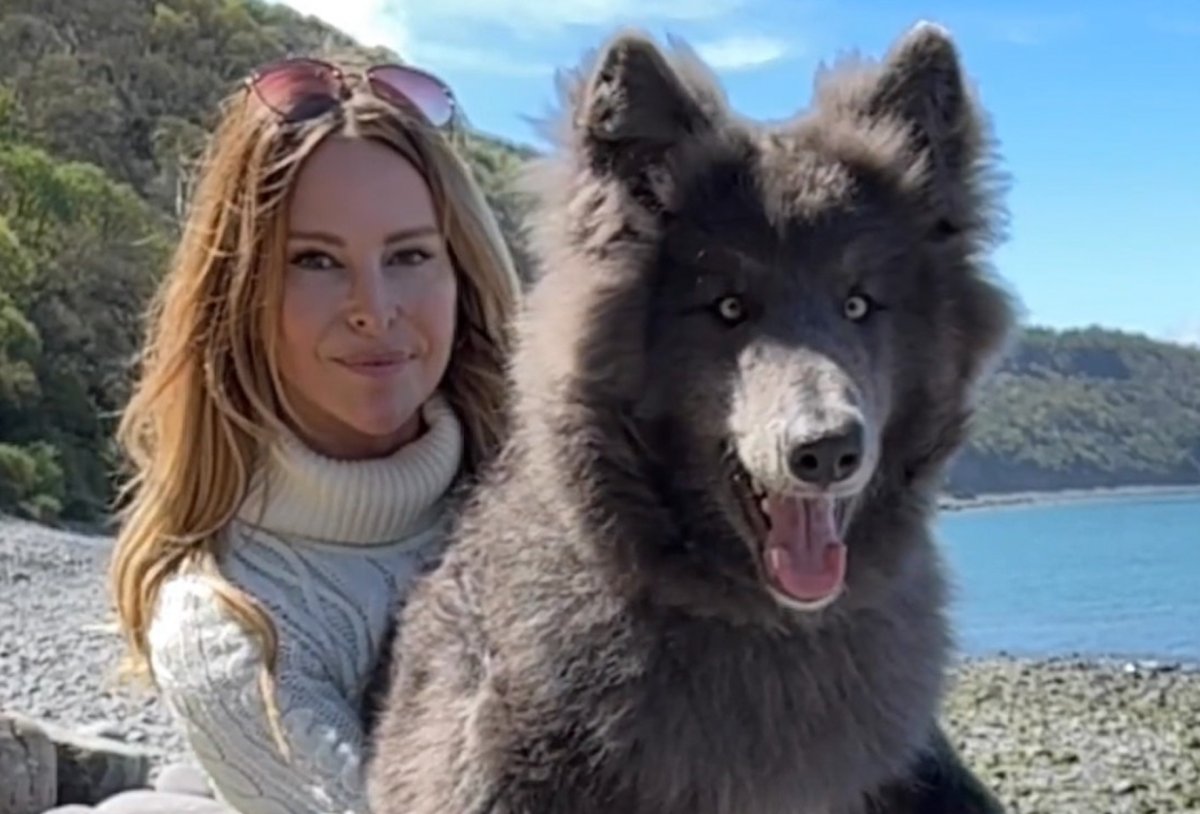**Descriptive Caption:**

In this vibrant daytime photograph taken at a scenic beach with hilly mountains in the background, a young woman in her mid-thirties is the focal point alongside her very large and fluffy gray and black dog. Adorned in a white knitted turtleneck sweater and wearing pink-tinted aviator sunglasses perched on her head, she stands out with her long, brunette hair cascading down. Her subtle, blush-colored lipstick complements her friendly visage as she gazes directly into the camera with a gentle, toothless smile.

Beside her, and stealing a bit of the show, is her exuberant companion, a large, fluffy dog with cartoonish, cross-eyed expressions and perky ears pointing upward. The dog's dark nose contrasts with its fluffy coat, and its mouth is open in a pant, conveying pure joy. Interestingly, the dog's appearance might remind one of a wolf due to its striking yellow-beige eyes and majestic posture. 

Behind the duo, the landscape unfurls in a picturesque manner: blue water, indicative of either a lake or an ocean; a stony beach; and lush, tree-covered hills reaching up into a sky dotted with small, puffy white clouds. The image captures not only the beauty of the natural setting but also the heartwarming bond between the woman and her furry friend.